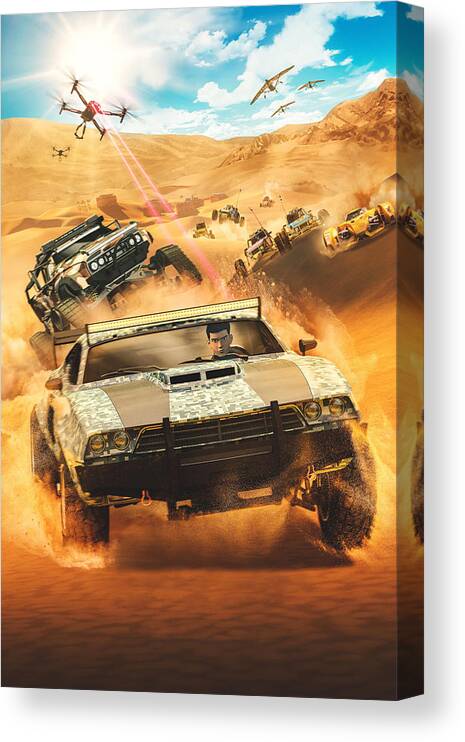The image showcases an intense scene from a video game set in a vast, arid desert landscape. In the background, towering mountains rise above rolling sand dunes, creating a dramatic, sunlit setting. The sky is a brilliant blue, dotted with fluffy clouds and a radiant sun glowing on the left side of the frame, casting its bright light over the scene.

In the foreground, a convoy of rugged, desert-adapted vehicles with large, robust wheels charges towards the camera, kicking up clouds of dust. The cars are camouflaged to blend in with the sandy environment, suggesting their purpose-built design for desert terrain. At the head of the convoy is a car driven by a focused man with black hair, his expression one of intense concentration.

In the background, more vehicles can be seen, trailing behind the lead car. Hovering in the sky above the convoy are several menacing drone-like machines, equipped with spinning propeller blades and emitting vivid red laser beams. These drones add a sense of urgency and danger to the scene. Additionally, three yellow aircraft hover on the right side of the image, contributing to the chaotic atmosphere of the scene.

The entire image is displayed on a thick canvas, adding a tangible, textured quality to the visual composition, with the canvas's thickness noticeable on the right-hand side.